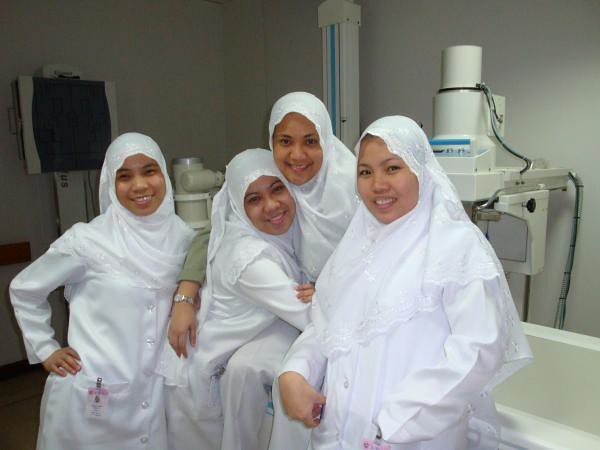This color photograph features four smiling women, all with an olive-brown complexion, suggesting they might be Hispanic, Middle Eastern, or Asian. They are dressed in white uniforms and wear long, white veils that drape over their shoulders and extend to their backs, typical attire for nurses. The woman in the middle, distinguished by a visible green sleeve and wristwatch, has her arm around the second woman, who also wears a similar white uniform and head covering, with her hand on her hip. The woman second from the left has an ID badge clipped to her coat. The four women are standing next to each other, three leaning against a table while one sits on it, hugging another. In the background, various medical equipment is visible, including a tall, white cylindrical object, what appears to be a large sign against a gray wall, and possibly a white sink at the bottom right corner, suggesting a hospital or clinical setting.